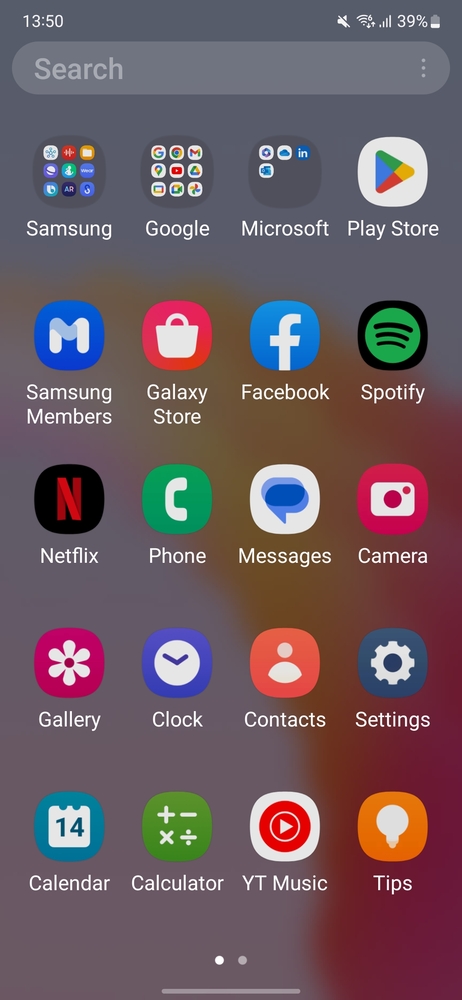This is a detailed screenshot of a smartphone homepage displaying various installed apps and system icons. At the top left, the current time is shown as 13:50. To the right of the time, there are status icons indicating sound, Wi-Fi connectivity, and the battery level, which is at 39%. Below these, there is a search bar with an icon of three vertical dots on the right side.

The homepage is organized with several app icons clearly visible, including:
- Samsung Apps folder
- Google Apps folder
- Microsoft Apps folder
- Google Play Store
- Samsung Members
- Galaxy Store
- Facebook
- Spotify
- Netflix
- Phone
- Messages
- Camera
- Gallery
- Clock
- Contacts
- Settings
- Calendar
- Calculator
- YouTube Music
- Tips

Overall, this screenshot provides a comprehensive overview of the phone's homepage and its functionalities, showcasing the wide array of applications available for use.